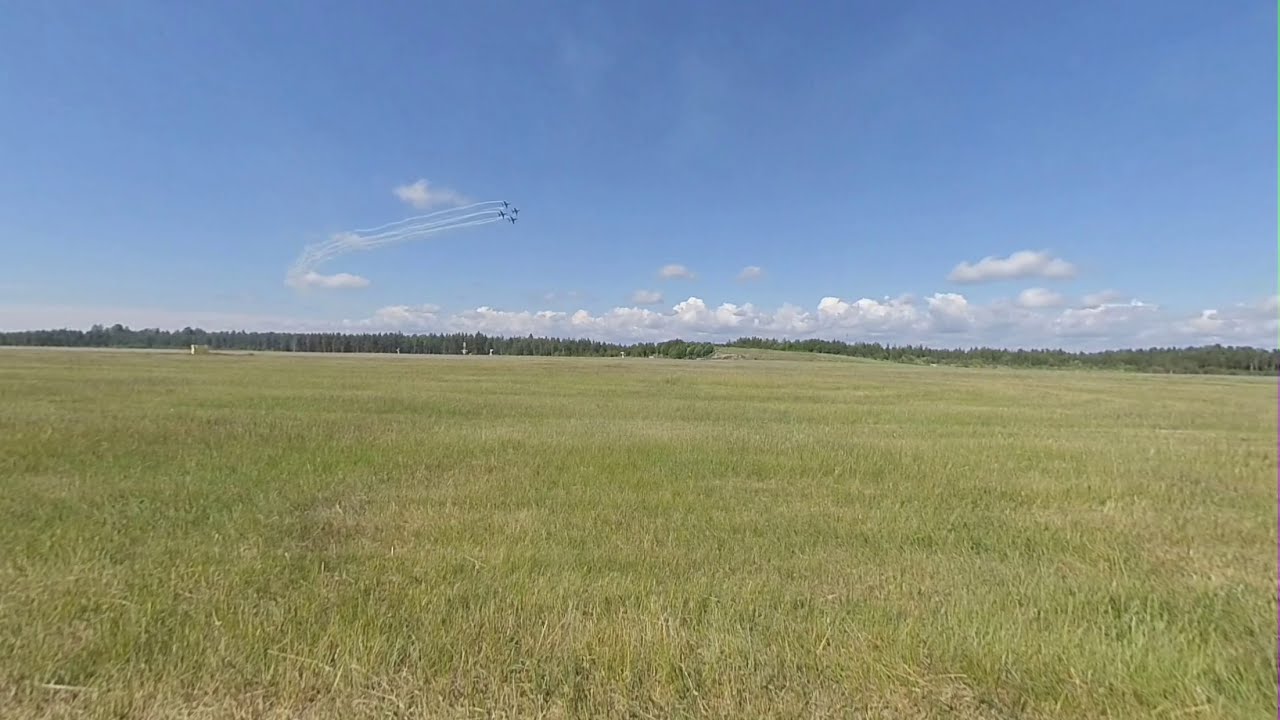The image shows a vast, slightly faded green grass field interspersed with touches of beige, giving it a uniform but subtly varied texture. The field stretches across the bottom half of the image. Towards the horizon, a row of dark green trees forms a continuous line, adding a sense of depth. Above this line of trees, a pale blue sky dominates the upper half of the image, gradually deepening in color towards the top. A few small puffs of white clouds hover above the horizon, contrasting with the predominantly blue sky. In the distance to the left, there's a barely discernible small white structure, adding a hint of human presence. Prominently visible in the sky are four jets, leaving contrails behind them, seemingly performing an aerial display. They are arranged in a diamond formation with one at the top, two on the sides, and another parallel to the first. Their white trails draw lines across the sky, converging towards the right side of the image.